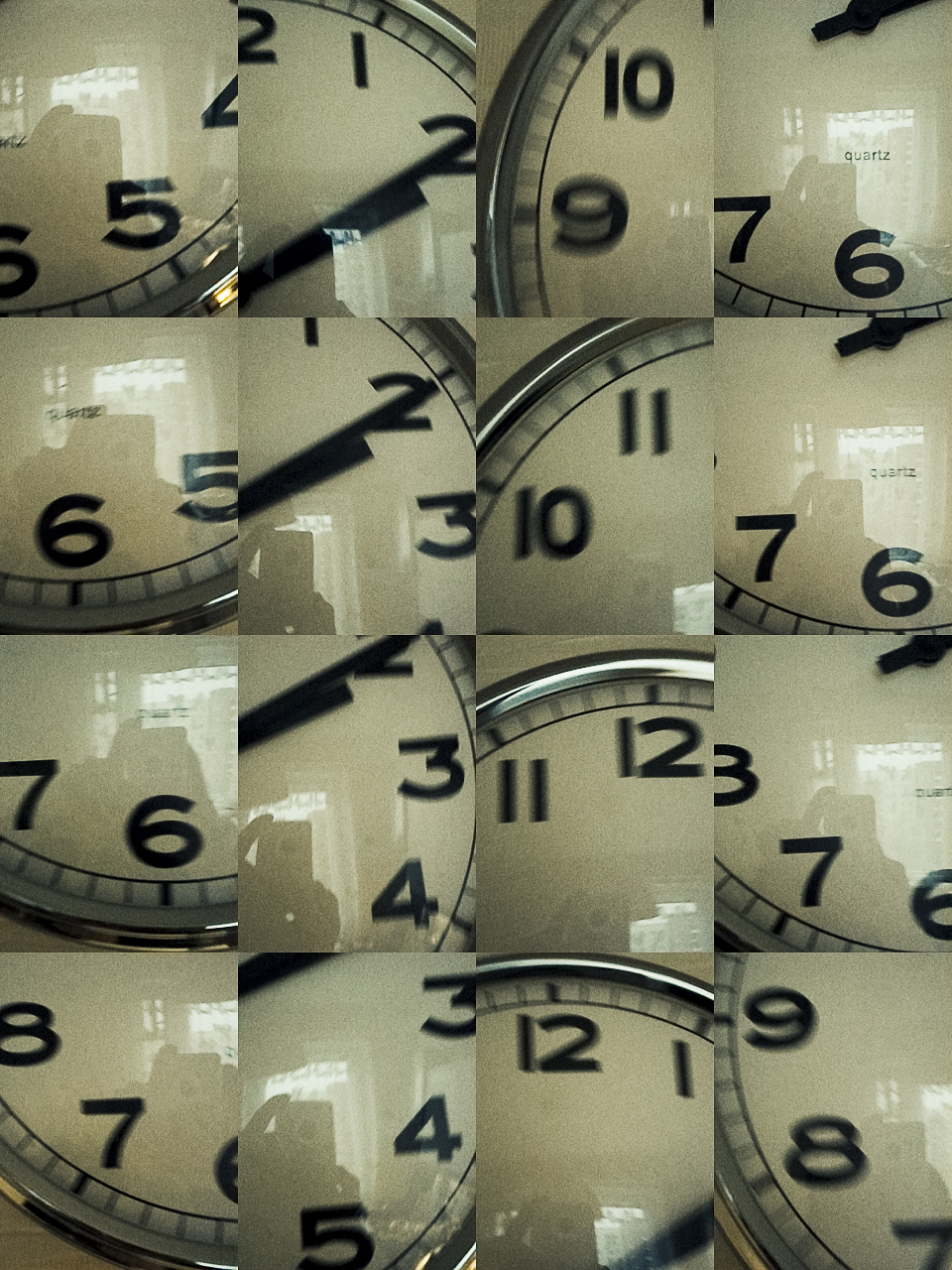The image depicts a composite of 16 closely zoomed-in photographs, arranged in a 4x4 grid, each focusing on different sections of a traditional analog clock face. Every photograph in this composite showcases a segment of the clock's numbers and hands, creating a detailed and meticulous mosaic of the clock's entirety. The sequence follows a pattern, with each row capturing segments of adjacent numbers and clock hands. For instance, the first column transitions from the area around the 6 to the 7, then to 7-6, and finally from the 8-7 segment. Similarly, the second column displays a sequence starting from around 12-1 to 2-3, and so forth. The clock face, characterized by its reflective glass or plastic cover, also reveals the faint reflection of the photographer holding a smartphone, with additional reflections suggesting the presence of a lit doorway behind them. The clock features a silver border and visible dashes marking the numerals, and an inscription indicating it is a quartz clock.